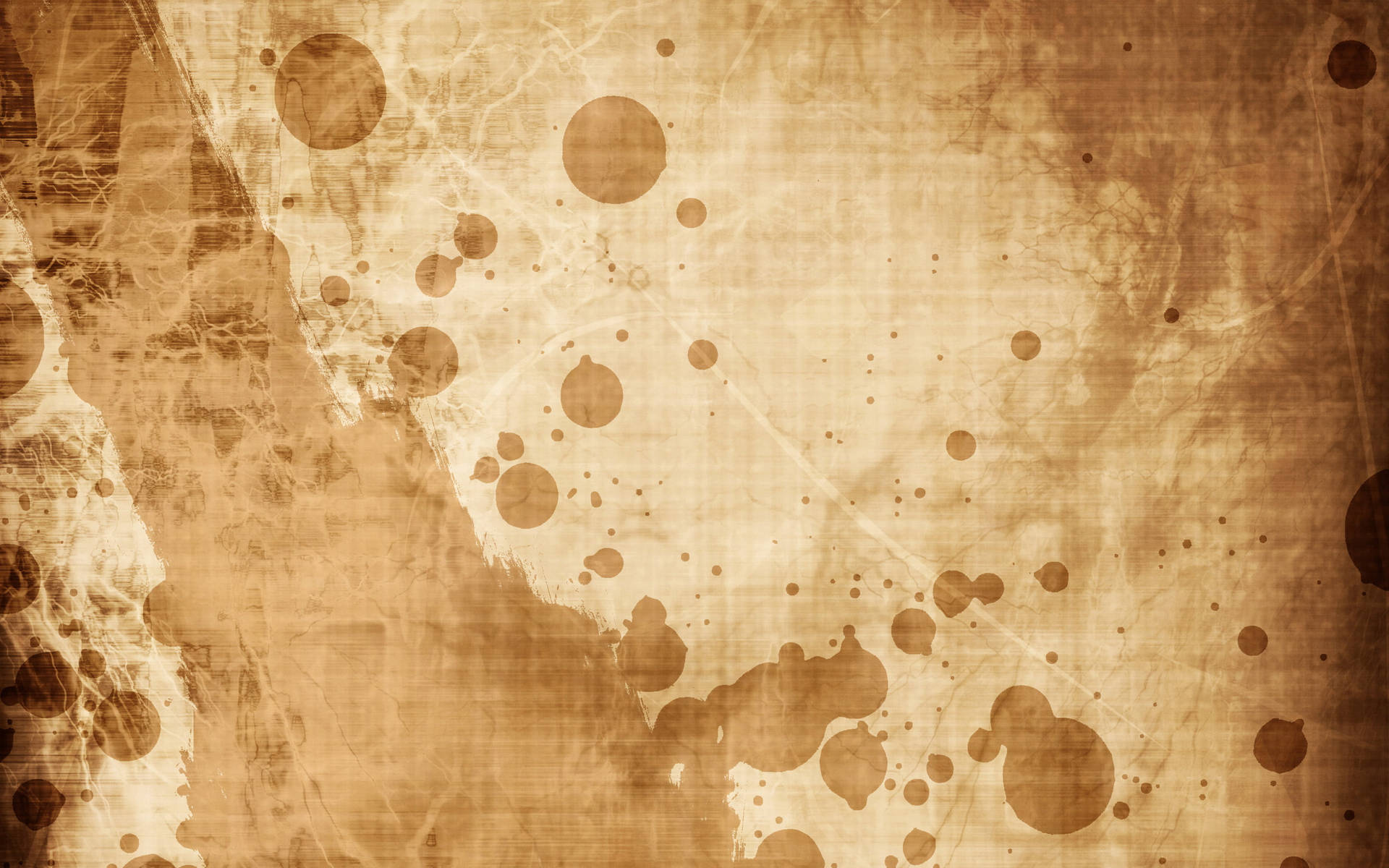This photograph captures a piece of fabric or paper that exudes an aged, distressed appearance. The surface is predominantly brown with a sepia tone, marked by various stains, dots, blotches, and splotches of differing sizes and shapes, resembling a tea-stained effect. The image is entirely filled by this textured material, presenting both lighter areas and a pronounced dark brown stripe that travels towards the left. Notable among the array of circular marks is a distinctive one featuring the visage of a man in profile, complete with glasses and a mustache, contributing to the artistic or possibly accidental design of the piece. The overall impression is that of an old, water-damaged item that might either be a photographically captured fabric, such as linen, or a digital rendering of such a distressed surface.